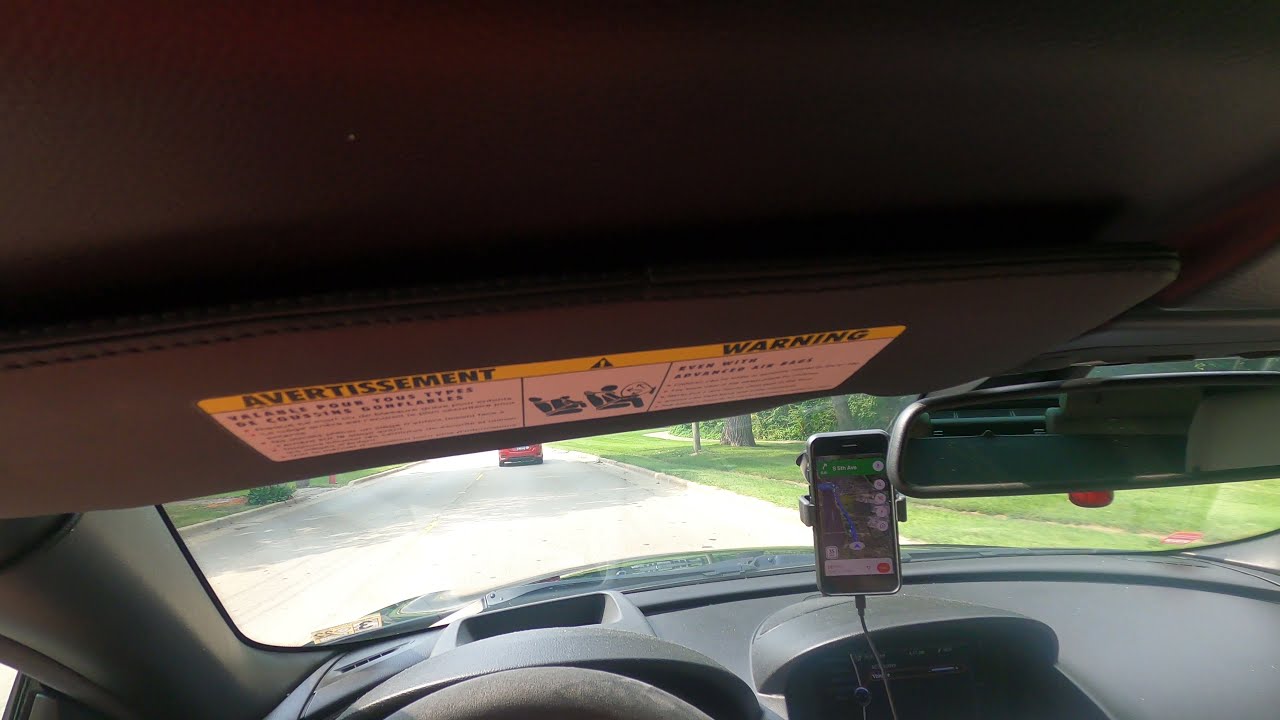The photograph, taken from inside a black car, captures a view from the driver's perspective looking out the windshield. The focus is primarily on the ceiling of the car, with the folded-up driver's side sun visor prominently visible. The visor features a sticker with sections labeled "advertisement" and "warning," with text in both French and English. To the right of the visor, you can see part of the rearview mirror. A cell phone is mounted on a holder that is suction-cupped to the windshield, displaying GPS navigation. Through the windshield, a wide road with well-mowed grassy curbs is visible. Ahead, the back of a red car can be seen, suggesting the photo was taken in a residential area with lush, green surroundings.